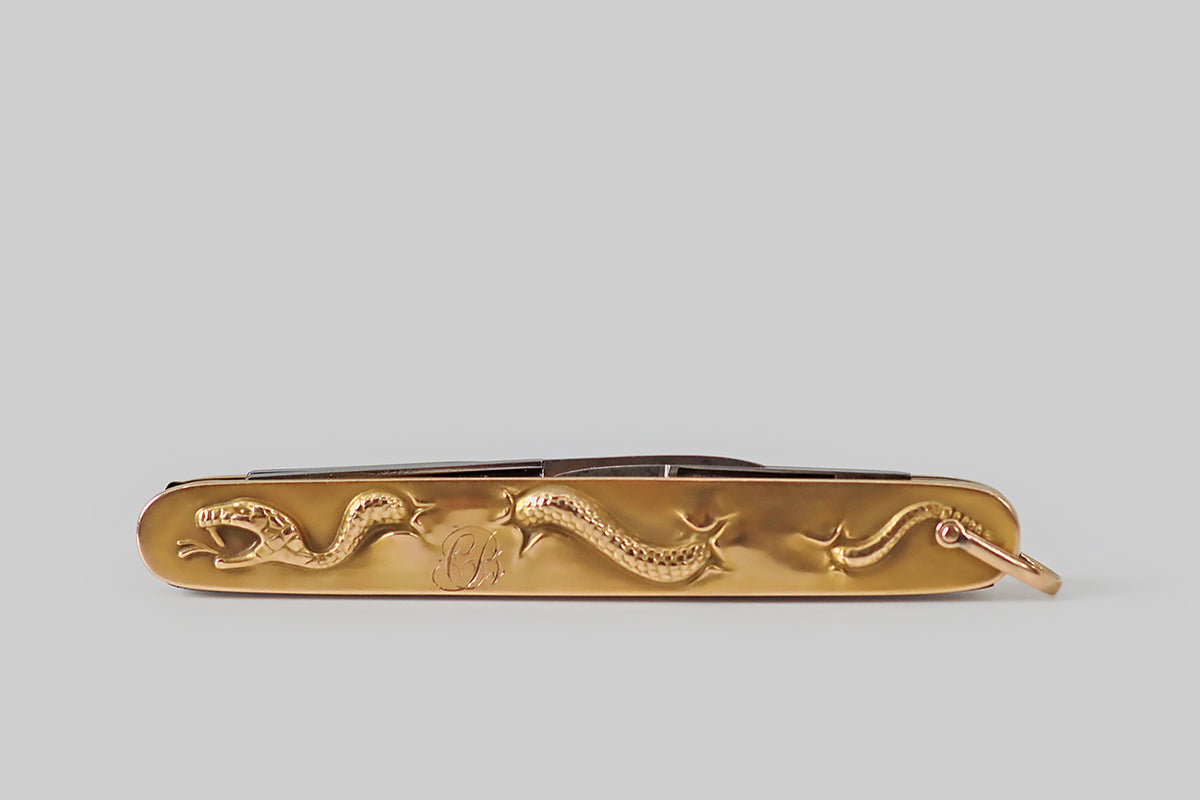A detailed, descriptive caption for the image:

"A gold penknife intricately designed with a serpent motif. The penknife features a single detailed serpent that winds sinuously from one side to the other. The snake, resembling a rattlesnake with noticeable fangs, appears to weave in and out of the metal surface, creating a striking visual effect. The serpent is not a bas-relief but rather sits proudly on the surface, showcasing meticulous craftsmanship. The gold penknife is of typical size and includes an attachment point for a keychain, enhancing its practicality. The serpent itself is rendered with fine detailing, highlighting its scales and textured body, adding to the overall elegance and uniqueness of the piece."